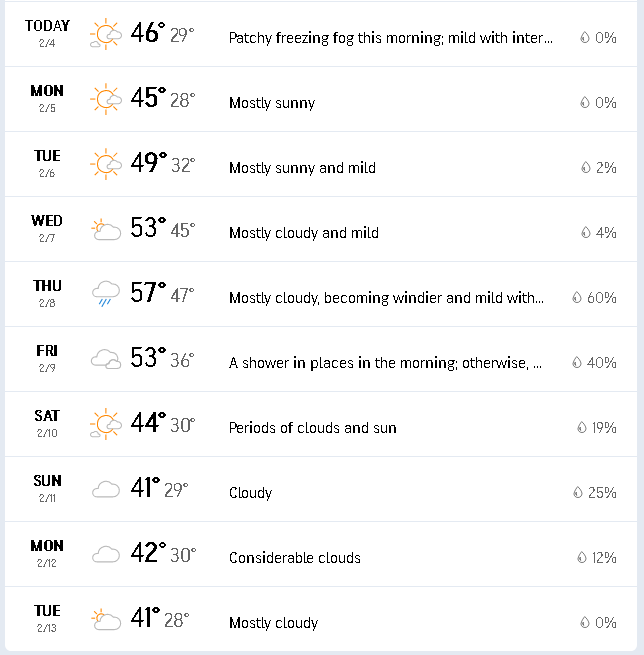The image displays a weather forecast spanning from February 4th to February 13th, presumably on a tablet or desktop screen due to its size, with temperatures shown in Fahrenheit. Here is the detailed weather forecast:

- **February 4th (Today):** Partly sunny with patchy freezing fog in the morning. High of 46°F and low of 29°F. 0% chance of precipitation.
- **February 5th (Monday):** Mostly sunny with a high of 45°F and a low of 28°F. 0% chance of precipitation.
- **February 6th (Tuesday):** Mostly sunny and mild. High of 49°F and low of 32°F. 2% chance of precipitation.
- **February 7th (Wednesday):** Mostly cloudy with mild temperatures. High of 53°F and low of 45°F. 4% chance of precipitation.
- **February 8th (Thursday):** Cloudy with increasing wind and a high likelihood of rain. High of 57°F and low of 47°F. 60% chance of precipitation.
- **February 9th (Friday):** Mostly cloudy with morning showers. High of 53°F and low of 36°F. 40% chance of precipitation.
- **February 10th (Saturday):** Partly sunny with periods of clouds. High of 44°F and low of 30°F. 19% chance of precipitation.
- **February 11th (Sunday):** Cloudy skies. High of 41°F and low of 29°F. 25% chance of precipitation.
- **February 12th (Monday):** Considerable cloudiness. High of 42°F and low of 30°F. 12% chance of precipitation.
- **February 13th (Tuesday):** Mostly cloudy. High of 41°F and low of 28°F. 0% chance of precipitation.

Overall, the forecast provides detailed weather predictions for over a week, indicating varying conditions from sunny to cloudy days, with occasional rain and fog.